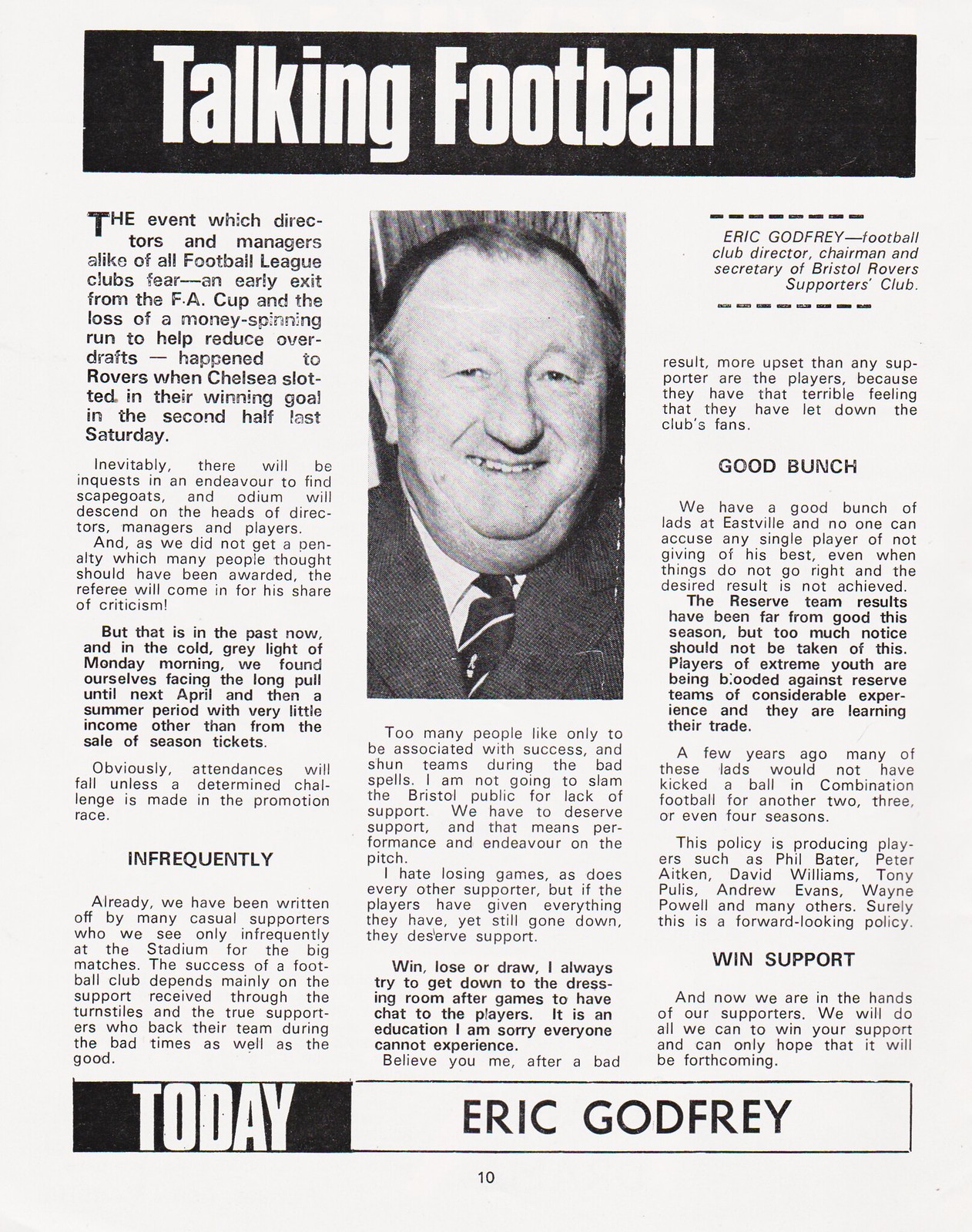This detailed newspaper or magazine clipping, labeled "Talking Football," appears to be an article featuring an interview with Eric Godfrey, who is the football club director, chairman, and secretary of the Bristol Rovers Supporters Club, a British athletic organization. The layout includes a striking top black bar spanning about a sixth of the page's height, with the title "Talking Football," and a thinner black and white bar at the bottom indicating "today" and "Eric Godfrey, page 10."

Central on the page is a close-up mugshot of Eric Godfrey, an older gentleman in his mid to late 60s, characterized by his short black hair, a slightly crooked smile, a large pointed nose, and a small ear. He is dressed formally in a black suit, black tie, and white shirt. The text is arranged in three distinct columns, segmented by subtitles such as "frequently," "good bunch," and "when support."

The article delves into the challenges faced by the Bristol Rovers following an early exit from the FA Cup due to a loss to Chelsea, leaving the club to contend with financial setbacks from missing out on a lucrative run. The discussion encapsulates the current state and future direction of the team, highlighting the financial strain faced in the interim period until the next season. The page, filled with straightforward newspaper-style printing, suggests an insightful read for those interested in the intricacies of football management and the personal reflections of Eric Godfrey.